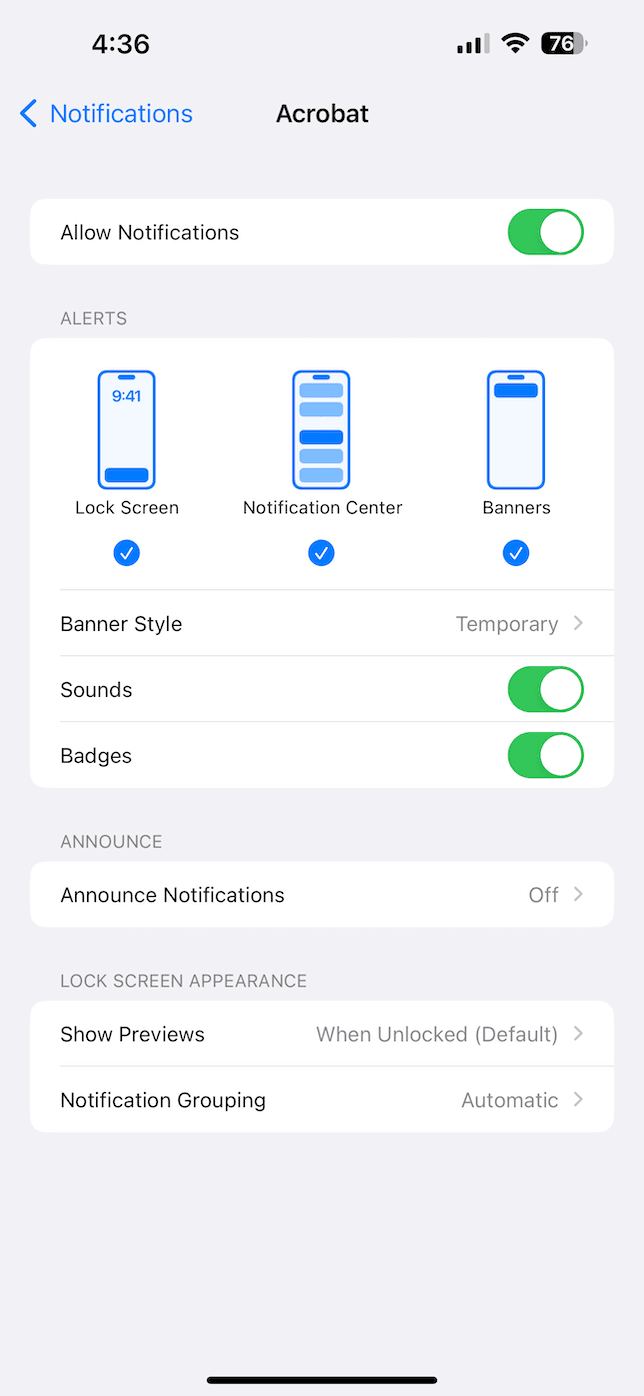Screenshot Caption: Apple iPhone Notification Settings for Acrobat App

This screenshot showcases the detailed notification settings for the Acrobat app on an Apple iOS device. The display is in System Settings, specifically under the Notification section. 

In the top-left corner, the time is visible, while the top-right corner shows the icons for signal strength, Wi-Fi, cellular connectivity, and battery level. 

Beneath the standard status bar, a blue-highlighted "Notifications" header is prominently visible, indicating the active settings menu. Next to this header on the left is a back arrow, and to its right, the app name "Acrobat" is displayed in black text.

The main portion of the screenshot displays various notification settings:

1. **Allow Notifications**: A white rectangular box with the text "Allow Notifications" on the left and a radio button on the right, which is turned on (green).
  
2. **Alerts**: Below the "Allow Notifications" setting, another white box provides options for different types of alerts.
    - Within this box, three icons represent the alert types: Lock Screen, Notification Center, and Banners. Each icon includes a blue checkbox underneath to indicate selection.

3. **Banner Style**: Three more rows define the style of the banner notifications.
    - To the right, it shows "Temporary" with a greater-than symbol (>) suggesting additional settings can be accessed.

4. **Sounds**: A radio button set to on (green) allows sound notifications.
  
5. **Badges**: A similar radio button enabled (green) for badge notifications.
  
6. **Announce Notifications**: Positioned below the badges, this setting has a white box indicating that "Announce Notifications" is turned off.
  
7. **Lock Screen Appearance**: This section includes two rows:
    - Show Previews: Set to "When Unlocked (Default)"
    - Notification Grouping: Set to "Automatic"

At the bottom of the screenshot, a thin gray bar stretches almost across the entire width of the display, marking the end of the settings options.